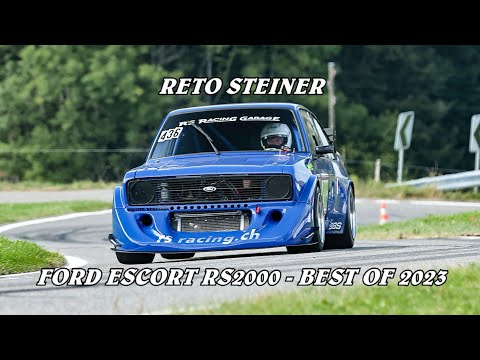The photograph showcases a light blue Ford Escort RS2000 with the number 436 prominently displayed and the text "Racing Garage" on its body. The image, reminiscent of the beginning of a YouTube video, features detailed white italicized text above and below the car, reading "Reto Steiner" and "Ford Escort RS2000 - Best of 2023" respectively, both with black outlines. The vehicle, appearing to lack visible headlights likely due to covers, is driven by a man wearing a white racing helmet with the visor up. The scene is set on a winding, green springtime road marked by guide rails, directional signs, and an orange cone to the right, suggesting a casual drive or a rally stage rather than an official racing track. The windshield bears the mark "RS Racing," and the front of the car displays "Racing.ch." The background is lush with bright green grass and trees, enhancing the vibrant, lively atmosphere of the setting.